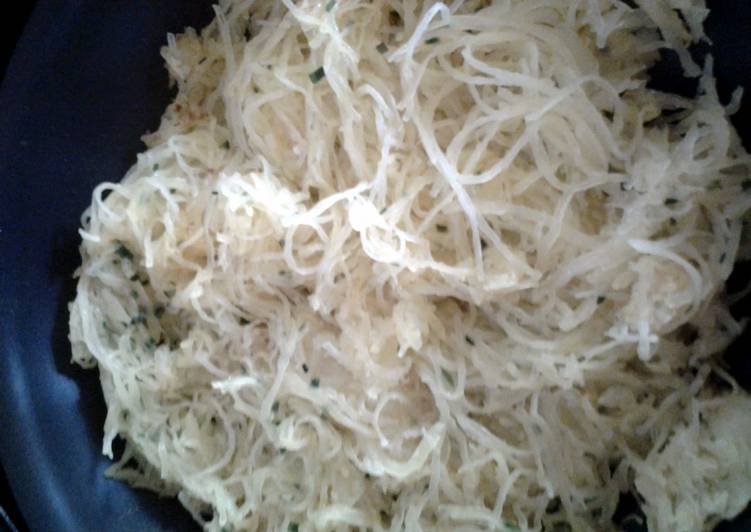The image depicts a close-up view of a plate of thin, white rice stick noodles, which appear slightly clumped together and sticky in texture. The plate, occupying most of the frame and positioned slightly to the right, is a dark navy blue color. The noodles have a stringy, pasta-like appearance and are garnished with green specks of onions or cilantro. The lighting is dim, suggesting the setting might be a kitchen or a dimly lit restaurant. Some of the noodles at the top left show a slight browning, indicating they are lightly fried or burnt. The overall visual impression is one of white, dense noodle strands intertwined with green garnishes on a contrasting dark plate.